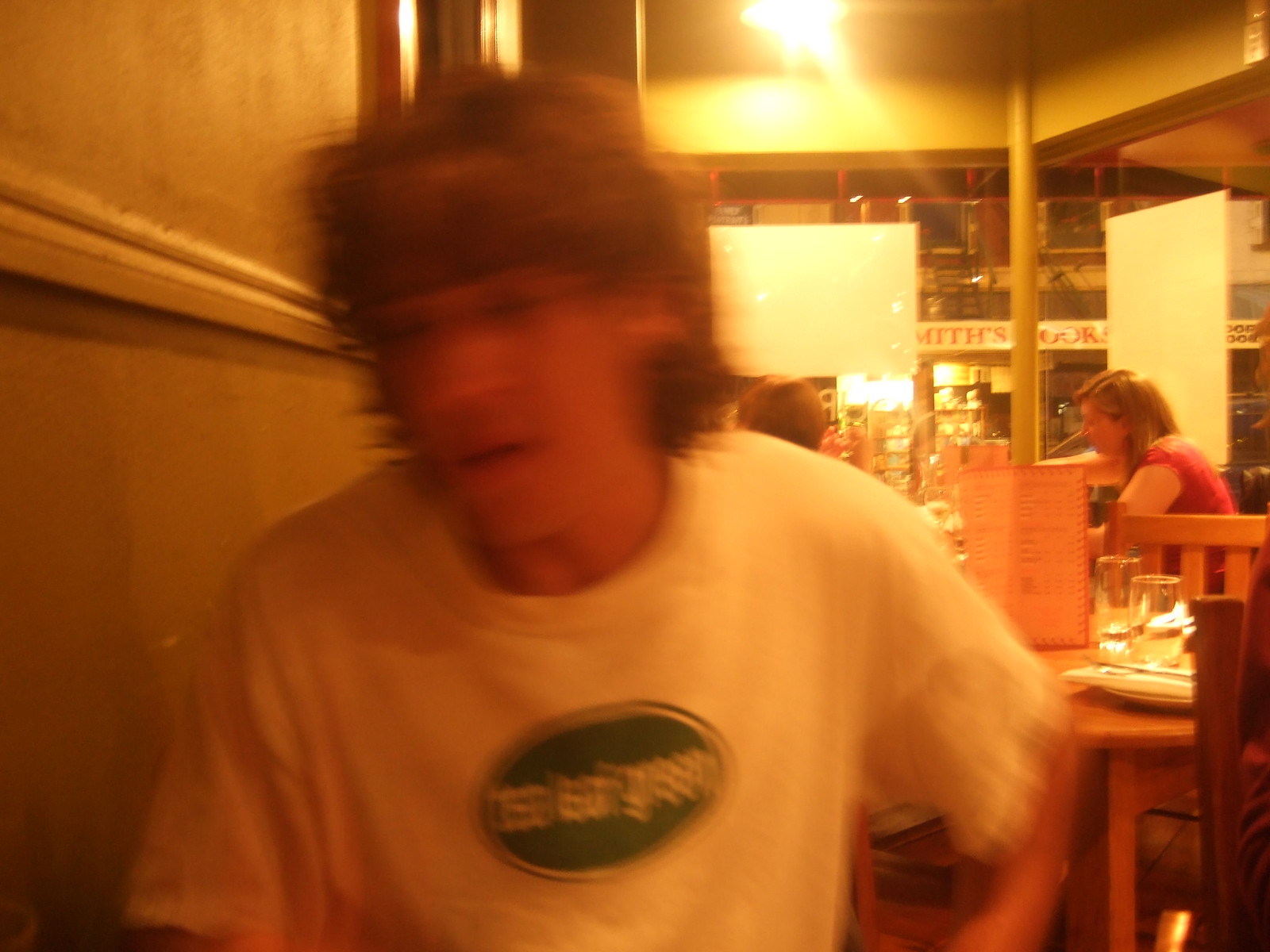In this somewhat blurred and yellow-tinted photo from the mid-2000s, the scene captures a bustling restaurant setting with a warm ambiance. A person, likely a man with long, shaggy brown hair reminiscent of Scooby-Doo's Shaggy, is foregrounded and appears to be looking down and to the right, their mouth slightly open. They are wearing a white T-shirt featuring a green oval logo with indistinct white text. The upper portion of the image is illuminated by a bright light, casting a red-tinted hue over parts of the scene. The left side of the photo is dominated by a wooden wall, and there are scattered dining tables below, topped with various dishes and glasses. Multiple patrons can be seen, including someone seated adjacent to a dining table with a vertically standing menu and another individual seemingly situated behind a bar area or another table. In the background, part of a sign reading "Smith's" is visible, partially obscured by objects and figures in the foreground. The overall setting suggests a lively, inviting restaurant environment.